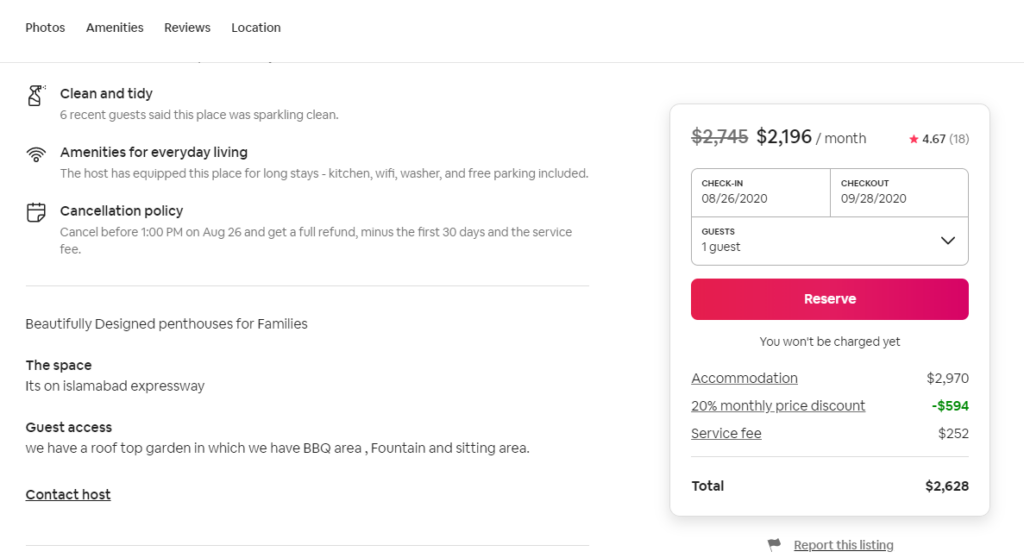**Image Description: Detailed Information of a Penthouse Listing**

The screen capture showcases a listing page against a white background with predominantly black text. At the top, navigational tabs read: **Photos, Amenities, Reviews, and Location**.

**Left Side Content:**

- **Subtitle**: Clean and Tidy
  - **Icon**: Spray bottle
  - Six recent guests have rated the place as sparkling clean.

- **Subtitle**: Amenities for Everyday Living
  - **Icon**: Wi-fi symbol
  - The host has equipped this place for long stays. Amenities include a kitchen, wi-fi, washer, and free parking.

- **Section**: Cancellation Policy
  - **Icon**: Calendar
  - Guests can cancel before 1 PM on August 26th for a full refund, minus the first 30 days and the service fee.

- **Highlight**: Beautifully Developed Penthouses for Families
  - **Location**: ISLAMABAD, Lomaspad, Espresso Way
  
- **Section**: Guest Access
  - The property features a rooftop garden equipped with a barbecue area, fountain, and sitting area.

- **Contact Information**: An option to contact the host is available.

**Right Side Content:**

- **Pricing Information**:
  - **Original Price**: $2,745 (crossed out)
  - **Discounted Price**: $2,196 per month
  - **Rating**: 4.67 stars from 18 reviews

- **Booking Details**:
  - **Check-in**: August 26, 2020
  - **Check-out**: September 28, 2020
  - **Guests**: 1 guest (selectable dropdown)

- **Reservation Box**:
  - **Button**: Pinky-red box labeled **Reserve**
  - **Note**: You won’t be charged yet.

- **Price Breakdown**:
  - **Accommodation**: $2,970
  - **Monthly Price Discount**: -$594 (in green)
  - **Service Fee**: $252
  - **Total**: $2,628

- **Icon**: Flag icon labeled **Report this listing**.

This screen capture provides a comprehensive overview of a penthouse listing, detailing its amenities, guest reviews, booking conditions, and pricing.